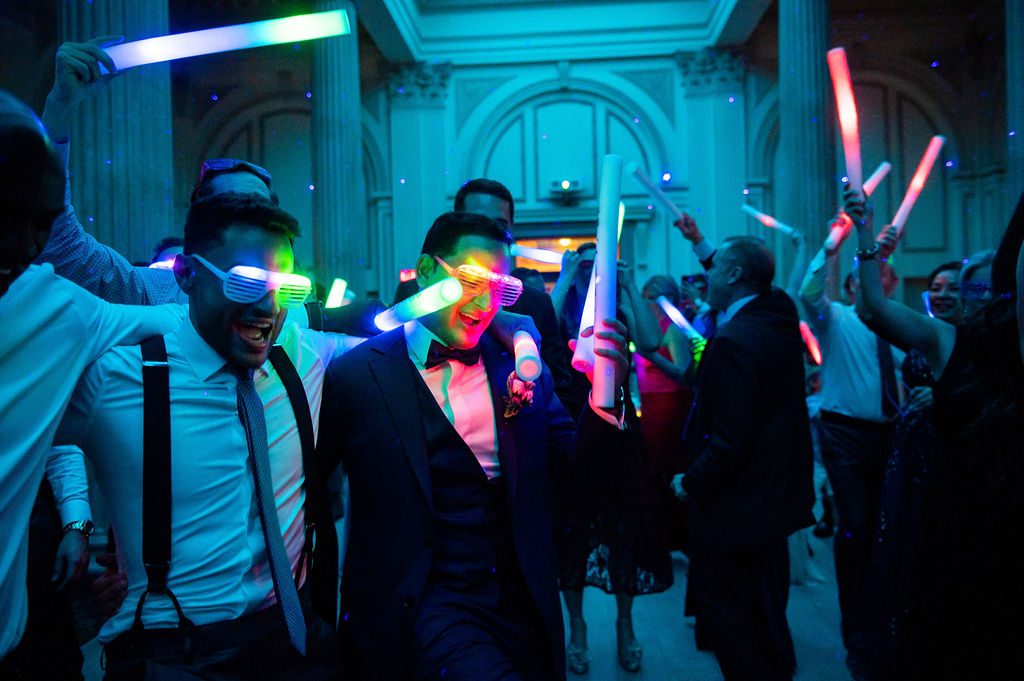The photograph captures a lively party set in a large building with white columns supporting a second story, suggesting a grand venue possibly for a New Year's celebration or a wedding. The guests are formally dressed, with most men wearing white shirts, black jackets, bow ties, or long ties paired with suspenders, pointing to a black-tie affair. Prominently, there's a man in a tuxedo with a black bow tie and a white shirt, dancing joyfully with another man who has his arm around him. This might indicate the man in the tuxedo is a significant figure, potentially the groom if it's a wedding. 

The atmosphere is vibrant, characterized by guests dancing and waving around multi-colored light-up tubes in shades of blue, green, red, and orange. These illuminate the darker room, casting an energetically festive mood. Some attendees on the left side sport distinctive vented, illuminated sunglasses, reminiscent of a playful, stylish touch. Despite the monochromatic appearance due to intense blue lighting, a sense of joy and celebration permeates the image as everyone smiles and enjoys the festivity.